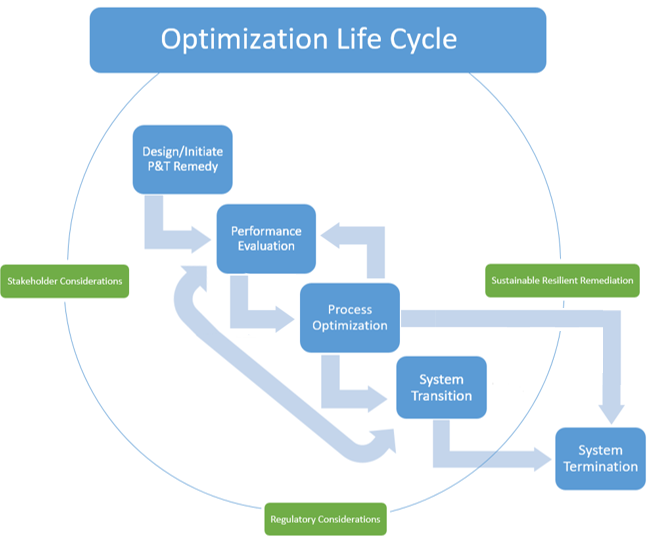This is an infographic titled "Optimization Lifecycle," prominently displayed in white text within a blue banner at the top. Below this title, a thin blue circle encloses five blue rectangles, each connected by arrows to illustrate a sequential flow from the top left to the bottom right. The first rectangle, labeled "Design/Initiate P&T Remedy," leads to "Performance Evaluation," then to "Process Optimization." This third rectangle has three arrows: one loops back to "Performance Evaluation," another proceeds to "System Transition," and a final one travels directly to "System Termination," which is situated outside the blue circle. Additionally, "System Transition" has a two-way arrow connecting back to "Performance Evaluation." Surrounding the blue circle are green rectangles labeled "Stakeholder Considerations" on the left, "Regulatory Considerations" at the bottom, and "Sustainable Resilient Remediation" on the right. This detailed illustration emphasizes the interconnected steps and considerations within the optimization lifecycle.